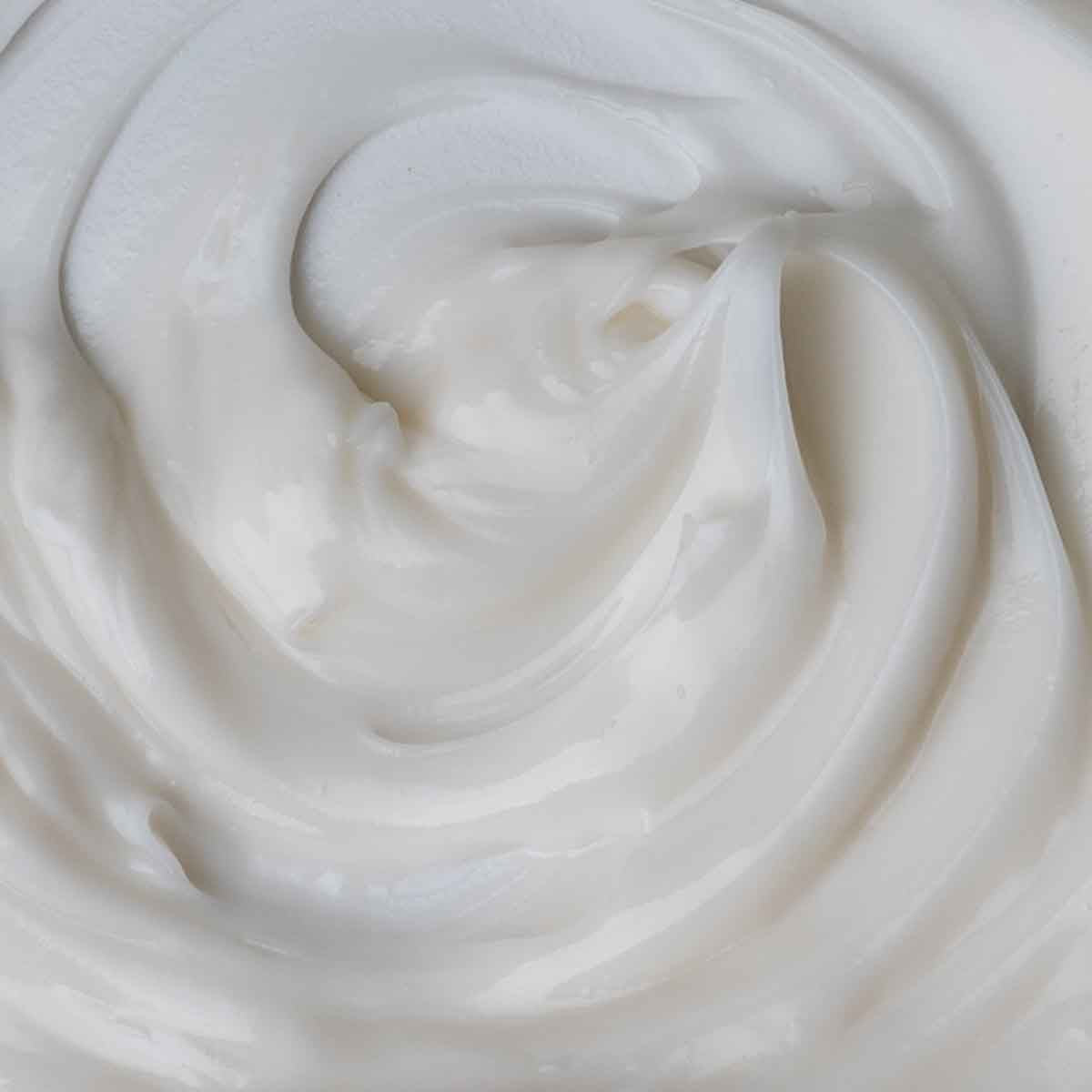The photograph is a detailed, close-up image of a white creamy substance, likely whipped cream, given its smooth, satiny, and shiny texture. The cream is semi-swirled, indicating it has recently been stirred, and you can see the distinct area where a spoon was lifted out. The whipped cream occupies the entirety of the frame, with no background, text, or color present. The ridges of some stiffer bands of the cream catch the light, adding to the sheen and making it appear freshly whipped. The high-quality image, likely captured with a modern camera or cellphone, resembles those used in advertisements, though devoid of any specific context or labeling, leaving the exact use or setting of the cream open to interpretation.